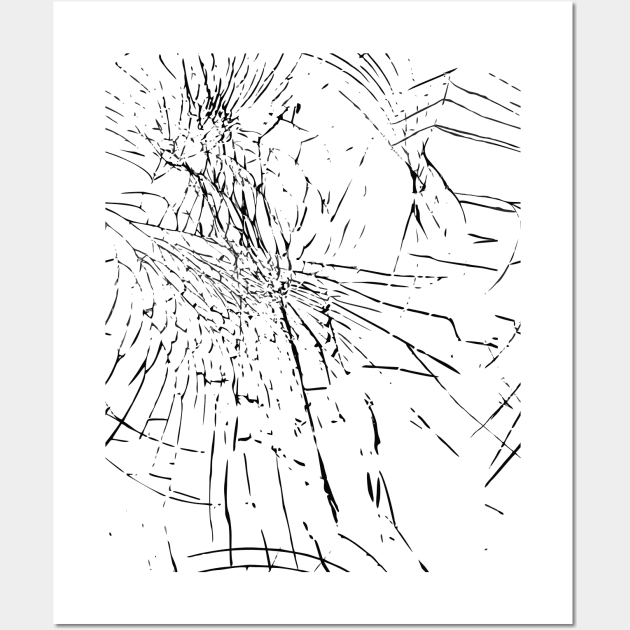This image is a black-and-white hand-drawn composition on a predominantly white canvas. The artwork consists of an array of black lines and strokes of varying lengths and directions, spanning the entire surface. These lines crisscross, curve, and intersect without forming any discernible pattern or shape. Notable elements include a section in the top right corner that resembles a potential building structure and another area that vaguely mirrors a shattered windshield. Additionally, some viewers might see abstract forms, such as a wing-like structure or the beak of a bird. The piece exudes a chaotic, impressionistic vibe, reminiscent of modern gallery art. The background is matte gray, providing a subtle contrast to the stark black and white of the drawing.